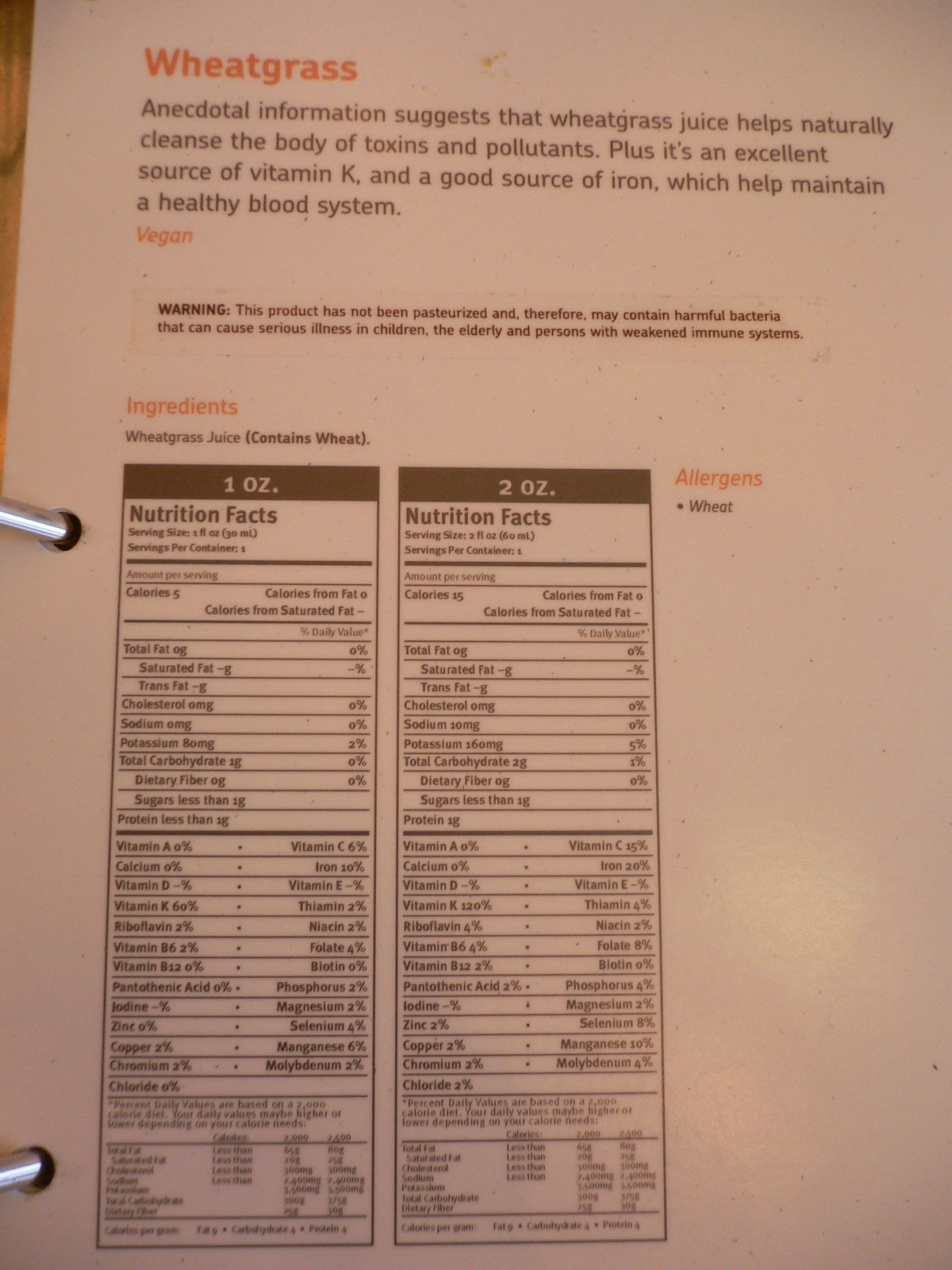At the top of the image, there is a section with an orange background containing text that reads, "Wheatgrass." Below that, it says, "Anecdotal information suggests that wheatgrass juice helps naturally cleanse the body of toxins and pollutants. Plus, it’s an excellent source of vitamin K and a good source of iron, which help maintain a healthy blood system." An orange label indicates it is vegan. Another warning in orange text states, "Warning: This product has not been pasteurized and therefore may contain harmful bacteria that can cause serious illness in children, the elderly, and persons with weak immune systems."

The ingredients list mentions wheatgrass juice, highlighting that it includes wheat. To the right, there is text about hygiene and taste, and to the left, it says "1 oz." Right next to it, "2 oz" is also mentioned. 

According to the nutrition facts for the 1 oz serving, it contains 5 calories. The details for the 2 oz serving reveal that it includes various vitamins, prominently mentioning vitamins A, K, D, among others. 

Overall, the label provides both nutritional benefits and necessary health warnings, ensuring consumers are well-informed about the product they are consuming.